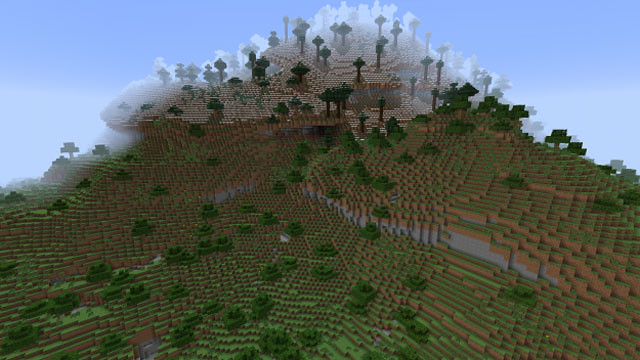This screenshot captures a scene from a Minecraft-style video game featuring a terraced, cube-like landscape stretching towards the top of the image. The terrain, reminiscent of Lego construction, comprises vivid green grass layers, interspersed with darker green trees and brown trunks, resembling green Lego pieces. The cubes' sides reveal layers of dirt and occasional gray patches, suggesting a tougher substratum. The scene ascends into a mountainous area with a distinctive white and gray haze, indicating incomplete processing or cloud cover. The summit is cloaked in this mist, behind which a light blue, cloudless sky unfurls. Towards the bottom left, a valley dips gently before the terrain rises again to form another slightly shorter peak on the right.